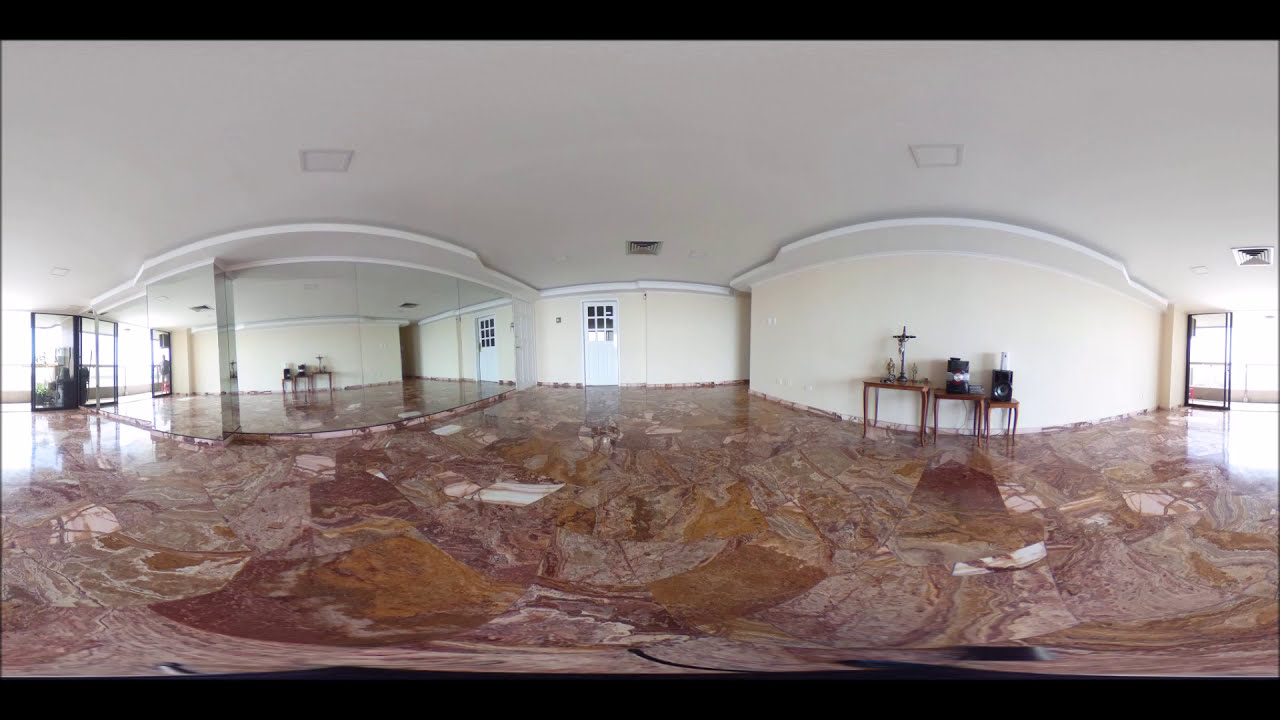The image depicts the interior of a large, spacious room that might be a posh hotel lobby or a religious church lobby. The room features an expansive, striking floor adorned with artistic mosaic tiles in a marble-like pattern of purples, browns, pinks, reds, and beige hues. The walls are an off-white to beige color, while the ceiling is white and features vents. On each end of the room are doors leading outside, with a prominent white front door at the center. Along one wall, which includes a mirror reflecting the opposite surfaces, there are small wooden tables in a copper brown color. These tables hold various items, such as a large decorative cross and a small speaker, adding subtle touches to the otherwise plain and clutter-free space. The overall atmosphere is one of elegance and tranquility, with no people present in the scene.